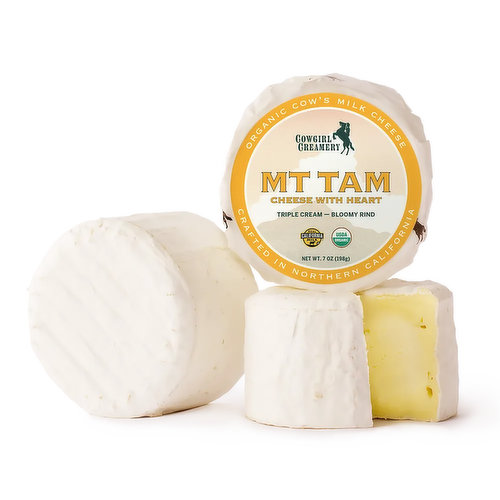The image features a close-up of three wheels of cheese, arranged to display both their exterior and interior, suggesting it's designed for advertisement purposes. The cheese is depicted with a white outer rind and a creamy yellow interior. The central focus is on the detailed label on the packaging. The label is edged with an orange ring that has white lettering stating "Organic Cow's Milk Cheese" at the top and "Crafted in Northern California" at the bottom. Inside this ring, against a lighter brown background, is the logo for Cowgirl Creamery, showcasing a rearing horse with a rider, presumably a cowgirl. Prominently in yellow letters, it reads "Mt Tam Cheese with Heart," and below that, in dark lettering, "Triple Cream Bloomy Rind." Additional smaller logos are visible, including one related to USDA approval, and a note indicating the net weight of seven ounces. One cheese wheel is shown on its side, displaying the top, while another is cut open to reveal its yellowish interior, emphasizing the creamy texture.